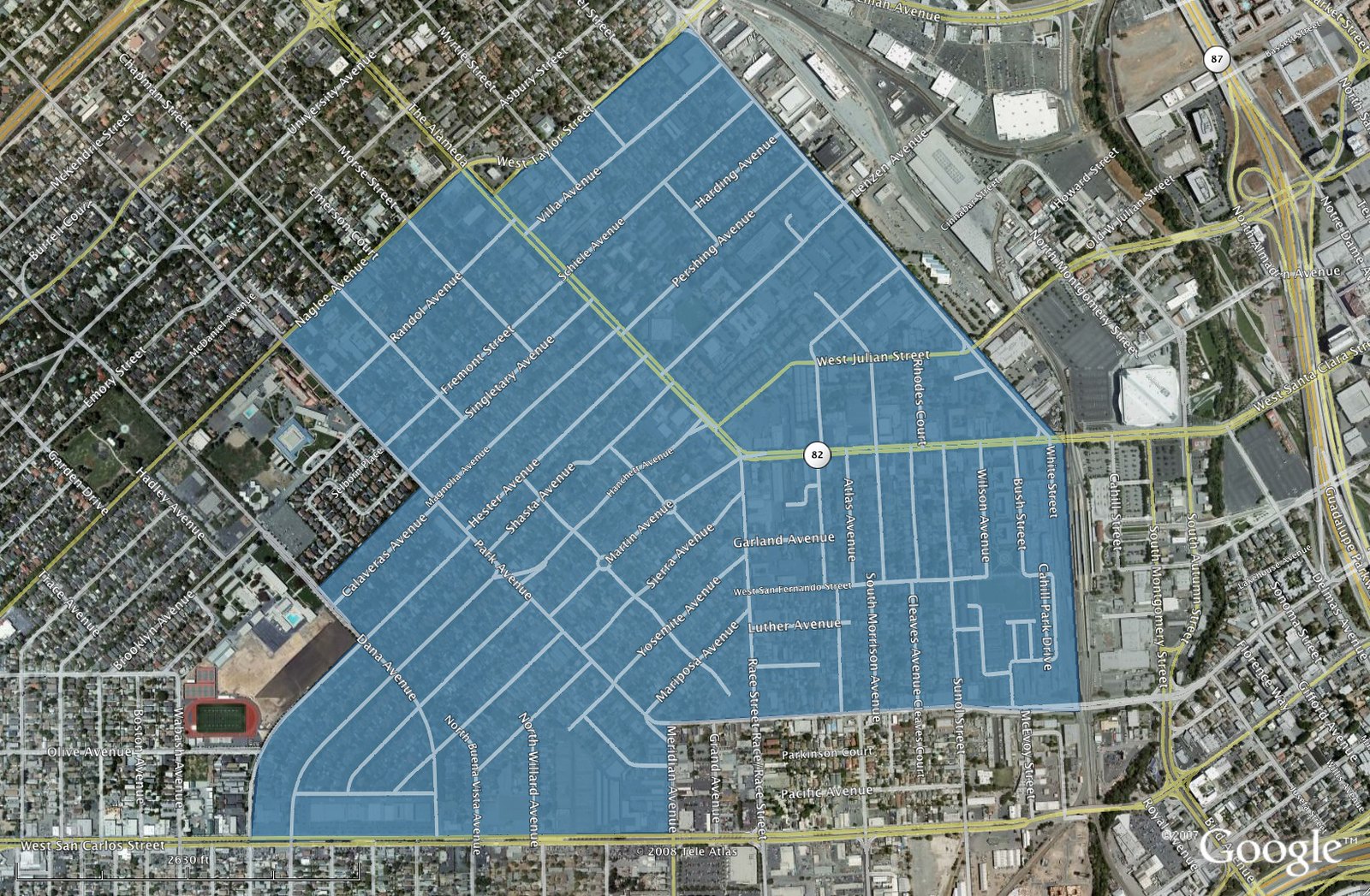The image depicts an overhead view of a densely populated urban area, captured in shades of blue, beige, yellow, brown, and gray, highlighting the city's grid-like structure. At the center lies a prominent blue area crisscrossed by lines representing highways. Surrounding this central grid are clusters of closely packed buildings and houses, predominantly dark-colored, interspersed with street and highway networks. The entire setting exudes a sense of congestion. The bottom of the image displays the distinct "Google" logo in white, indicating that this is a Google area map. Specific details about the city or individual buildings are indiscernible, but the overall layout suggests a bustling and crowded metropolis.